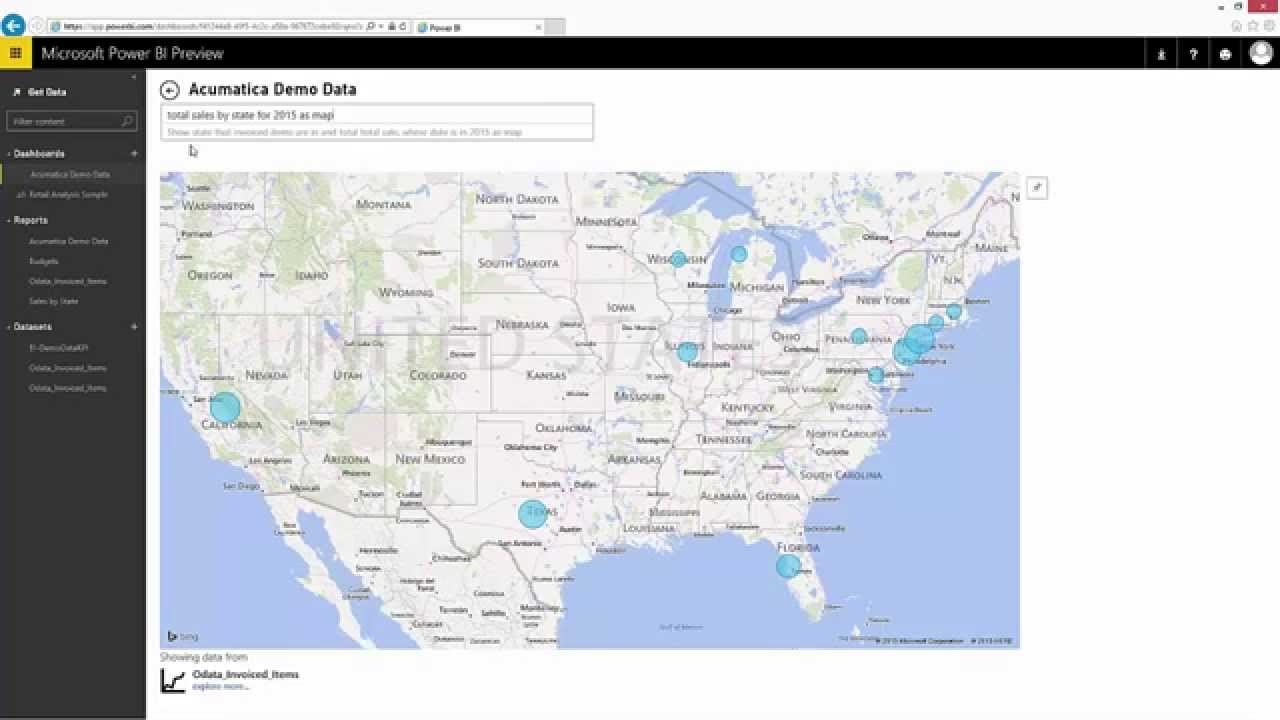The image showcases a website featuring a detailed map of the United States. At the top of the page, there is a white search bar set against a black border, which also extends thicker along the left side. The header includes the text "Acumatica demo data" with a white box positioned below it. Dominating the main section is a vividly illustrated map of the United States, complete with state names and geographical details, such as mountain ranges. Notably, the map displays several light blue bubbles dispersed throughout various regions, with a high concentration in the northeastern states like Pennsylvania, New York, and New Jersey, extending up the coastline through Connecticut. Additional bubbles are visible in the Midwest, Florida, Texas, and California. The bubbles likely contain specific information, although the text appears too faint to read clearly. Similarly, the left-side black border contains extensive text, which is small and difficult to decipher.